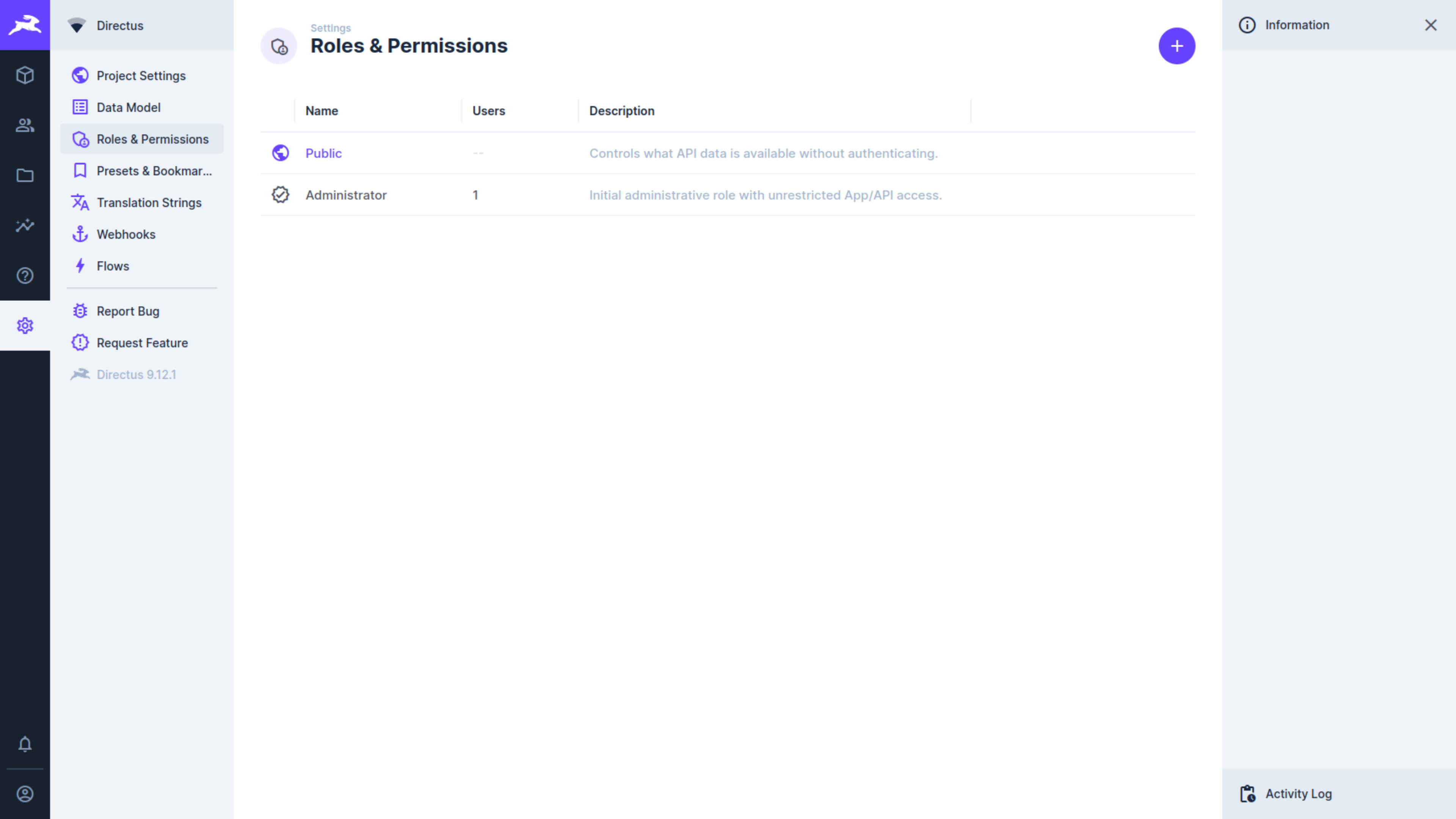The image depicts a comprehensive webpage interface designed for managing various project settings. On the left pane, there is a navigation menu featuring multiple sections including Directors, Project Settings, Data Model, Roles and Permissions, Presets and Bookmarks, Translation, Strings, Webhooks, Flows, Report Log, Request Future, and Roles and Permissions (listed a second time). Further down on the menu, specific options such as Name, Public, Users, and Description are visible. 

Detailed explanations are provided for several items:
- "Controls what API data is available without authenticating" suggests management of API data accessibility.
- "Administrator, Users" outlines the initial administrative role with unrestricted access to app or API assets.

On the right side of the interface, there is an information panel displaying detailed information and activity logs relevant to the selected items from the left pane. This dual-pane layout allows for seamless navigation and detailed inspection of project-specific configurations and settings.